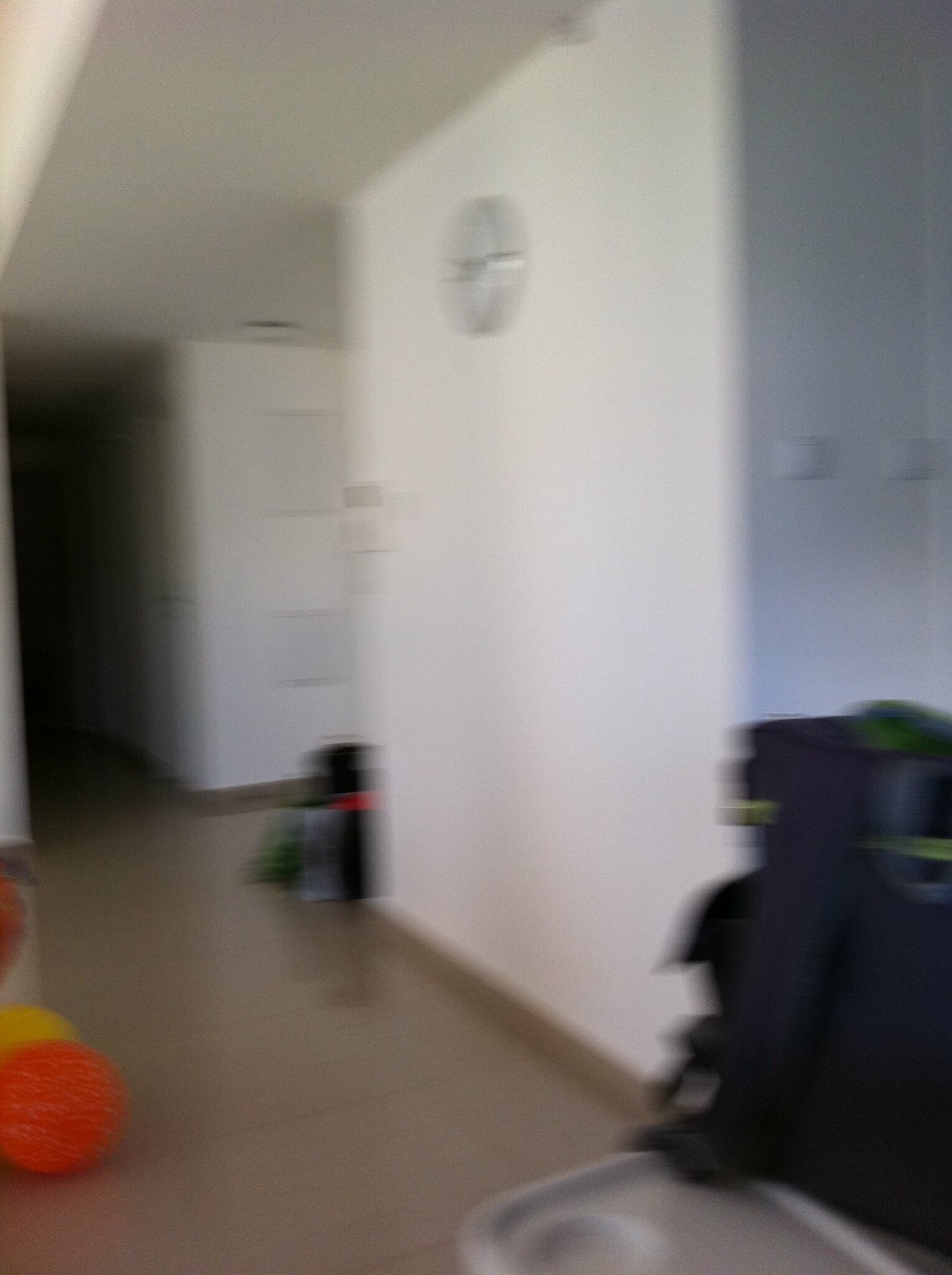This is a color photograph taken indoors, inside someone's home, and it displays a slightly blurry hallway scene with several visible details. The hallway features white walls adorned with light switches and a wall clock, although the hands on the clock are indistinct. The floor is covered in a brownish linoleum that extends throughout the home, accompanied by brown base trim. In the foreground, to the right of the image, we see some luggage or suitcases against the white wall. Among these items, there is something black with a red band and another object that appears gray or green-gray. Additionally, there's a black backpack-like item with a bit of green at the top, next to which a plastic tray is visible. On the bottom left corner, there's a toy with red and yellow wheels, alongside a textured orange ball in front of a yellow ball, each about the size of a basketball. Further down the hallway, there are more objects, possibly another set of luggage or backpacks, as well as a corridor leading to a dark area on the left and another hallway branching off to the right.